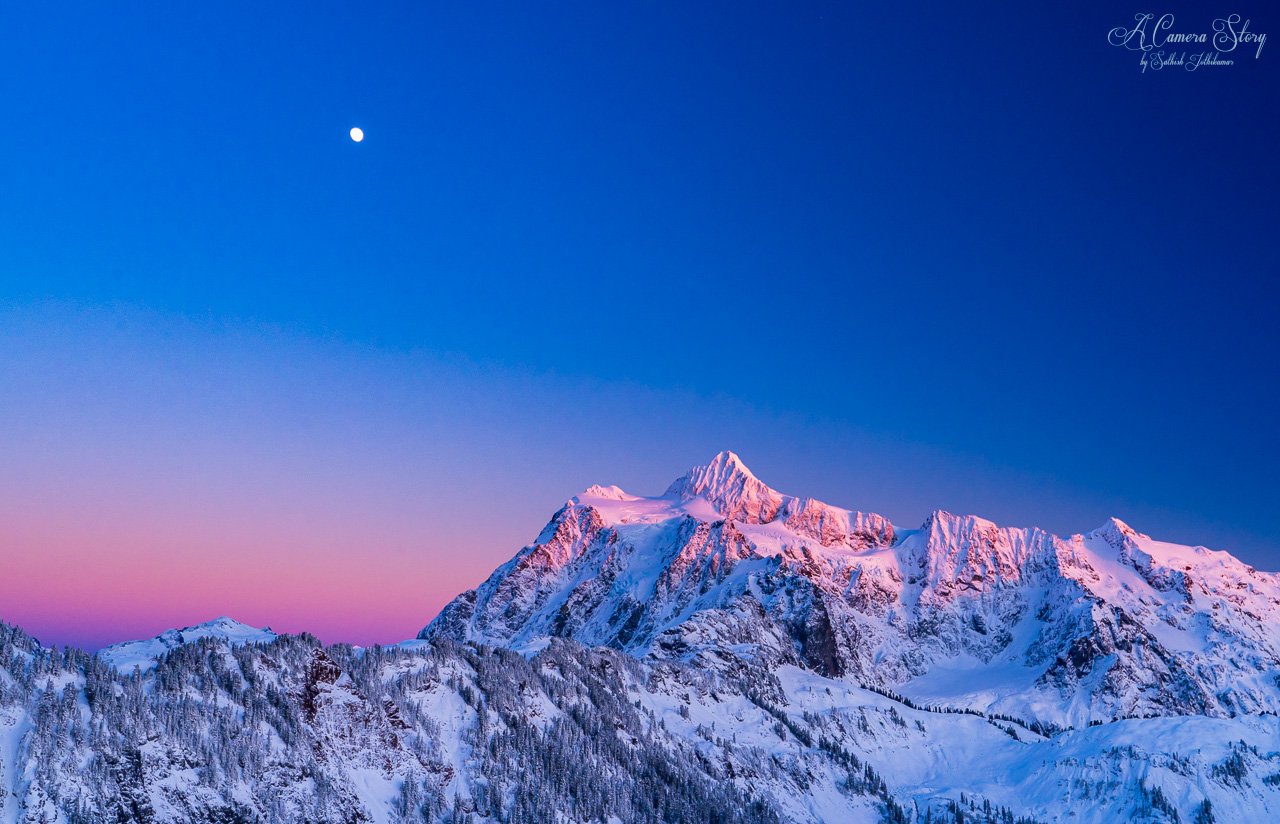This stunning color photograph captures a snow-covered mountainscape under a striking, clear sky. The image, taken almost at nighttime, features a high-contrast, saturated scene where the peaks, covered with fresh snow and dotted with pine trees, dominate the bottom half. The white snow glistens with a slight blue tint, enhancing the sense of peace and tranquility. The sky transitions beautifully from a dark royal blue at the top to a pinkish-orange gradient near the horizon, suggesting either a sunrise or sunset. Adding to the serene atmosphere, a tiny, circular white moon is visible in the top left corner, softly illuminating the scene. In the top right corner, in elegant cursive, is the watermark "A Camera Story by [Name] Johnson," attributing the artwork to its photographer.